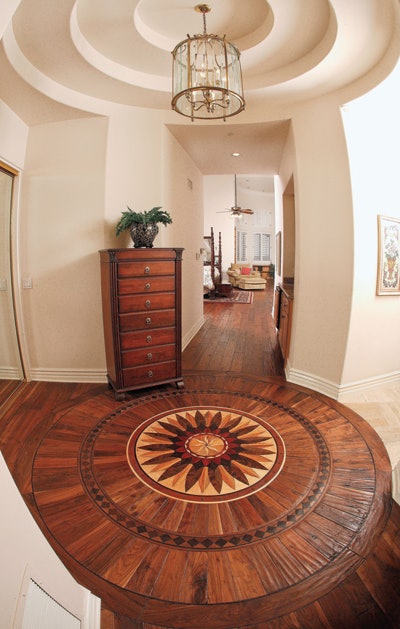This is a detailed interior photo of a residential home, specifically capturing an entry hallway and extending view into an adjacent room. The setting is indoors, photographed with a wide-angle lens that distorts and rounds the perspective. The hardwood floors stand out prominently, and a circular inlaid design dominates the entrance area. This medallion features concentric circles and sunburst-like protrusions, incorporating colors of white, brown, and yellow with an antique flower petal motif. 

Flanking the left side of the circular design is a wooden chest of eight drawers, each with a single central knob, topped with a gold and metal vase containing green plants. An ornate glass and gold chandelier hangs from a ceiling adorned with concentric circular details, mirroring the floor's motif.

To the right, a hallway leads to white walls adorned with a framed print of a plant. The background reveals an additional room featuring varied furnishings like a four-poster bed, an easy chair with a red and orange pillow, a recliner, an ottoman, and a ceiling fan. Large windows grant a glimpse of daylight, enhancing the room's airy feel. The entire home has a minimalist yet elegant decor, emphasizing understated design elements throughout.